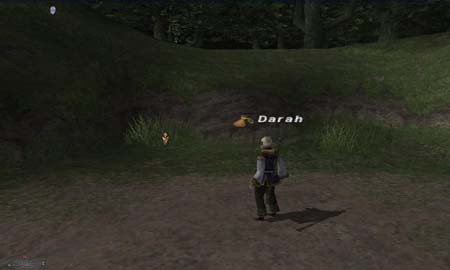In this screenshot from a video game, the image primarily features a single player character situated centrally in a landscape comprised of grass and sparse dirt patches. The scene is predominantly dark in tone, giving it a moody or evening ambiance. Surrounding the character are a few small green bushes adding a touch of nature to the scene.

The player's in-game name, "D.A.R.A.H.", is prominently displayed above the character in white text. To the immediate left of the name is a small, golden-colored symbol, possibly depicting a bag or another unspecified item.

The character is dressed in an outfit reminiscent of Odin-inspired fashion. The attire includes a flowing white shirt with long, loose, bell-shaped sleeves, while the remainder of the clothing is black, adding to the medieval or mystical theme of the game.